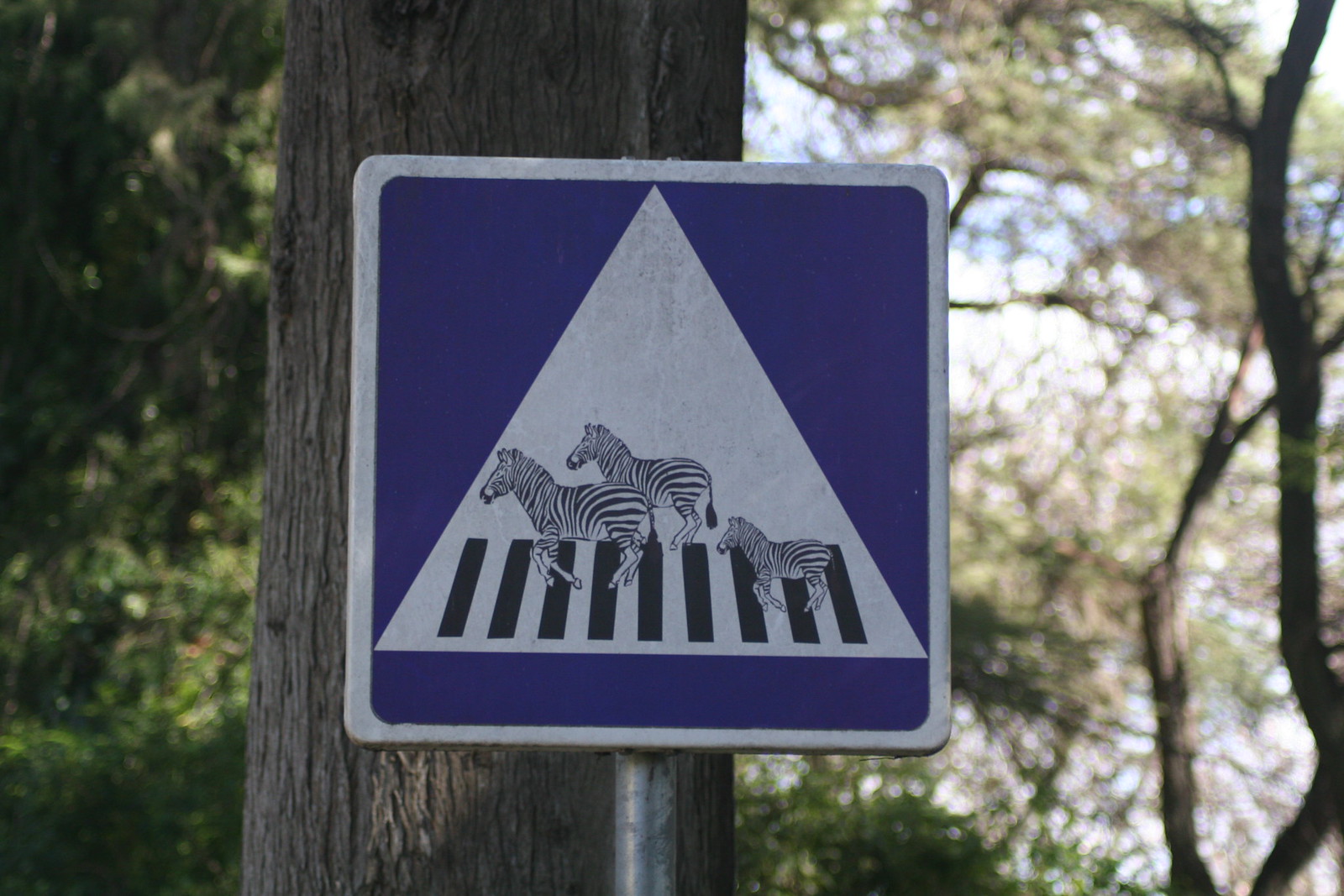The photograph captures a vivid street sign centered prominently in the image, mounted on a silver metal pole. The sign itself is square with rounded corners, featuring a vibrant blue background and a white border. Dominating the sign's design is a central white equilateral triangle displaying a meticulously detailed zebra crossing. The crossing is depicted with alternating black and white stripes resembling piano keys, and three zebras—two adults and one juvenile—are illustrated traversing from left to right, characterized by their distinctive black and white stripes.

Behind the sign, a slightly out-of-focus tree trunk is visible, with branches and an abundant canopy of leaves providing a shaded backdrop. Additional trees with leaves in varying shades of green are present in the background, some areas illuminated by sunlight filtering through the foliage. The sky peeks through the leaves, hinting at a bright day with partial cloud cover, further enhancing the ambiance of the scene.